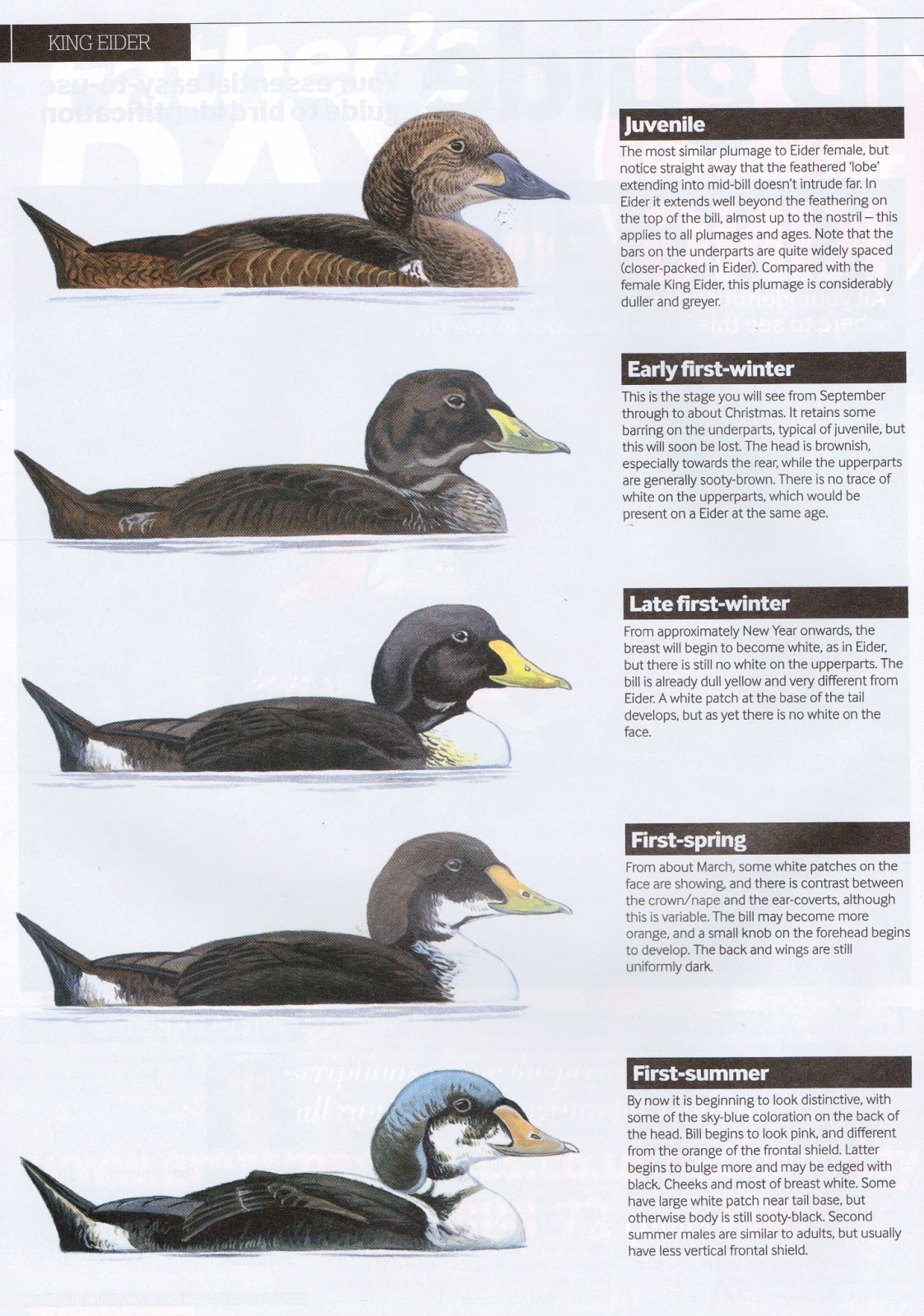The full-color, vertically rectangular artistic image features a detailed display illustrating the life stages of the King Eider duck. The background is a bluish off-white, adding a subtle contrast. At the top left corner, a black rectangle with white text reads "King Eider." Each developmental stage of the duck's life is presented in a sequence with corresponding images and informative paragraphs. 

The sequence begins with a "Juvenile" stage, showing a light brown duck. Following this is the "Early First Winter" stage, where the duck appears darker with details about this stage being from September to around Christmas. Next is the "Late First Winter" phase, depicting a primarily black duck with a bright yellow bill. As we move to "First Spring," the duck exhibits more white feathers and a slightly lighter bill. Finally, the "First Summer" stage shows the duck with a blue and green head, a more faded bill, and consistent feather coloration.

Each title for the stages—Juvenile, Early First Winter, Late First Winter, First Spring, and First Summer—is presented in white text within rectangular brown shapes, ensuring clarity and distinction of each life phase.